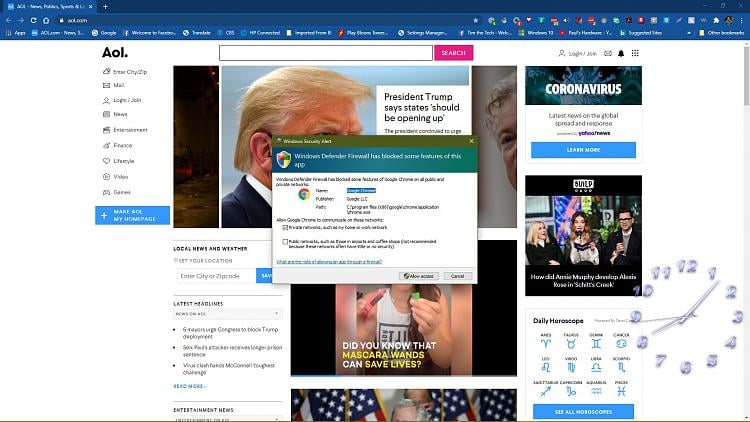This image features a web browser window with a darker blue banner at the top and several open tabs, the foremost one being labeled "AOL News." Adjacent to the open tab is a darker line containing a plus sign for adding new tabs. Moving downward, there is a toolbar with backward and forward navigation arrows, a refresh button, a home button, and a search/address bar displaying "AOL."

Below this toolbar is a row with quick access links labeled as "Apps," "AOL.com," "Google," "Welcome to Facebook," "HB Connected," and a few other indistinguishable ones. To the right of the address bar, a line of icons is visible.

The main portion of the browser displays the AOL homepage, which is predominantly white. At the top, "AOL" is prominently written in bold black print, accompanied by a search bar with a pink search button beside it. Below this are links to various sections such as "Mail," "Blog & Jewelry," "News," "Print," "Finance," "Lifestyle," "Video," and "Games." Additionally, there is an option to "Make AOL my homepage" accompanied by a plus sign.

A pop-up notification appears over the webpage, indicating that "Windows Defender Firewall has blocked some features of this app." The notification lists the app's name, the publisher, and the option to allow "Google Chrome to communicate on this network."